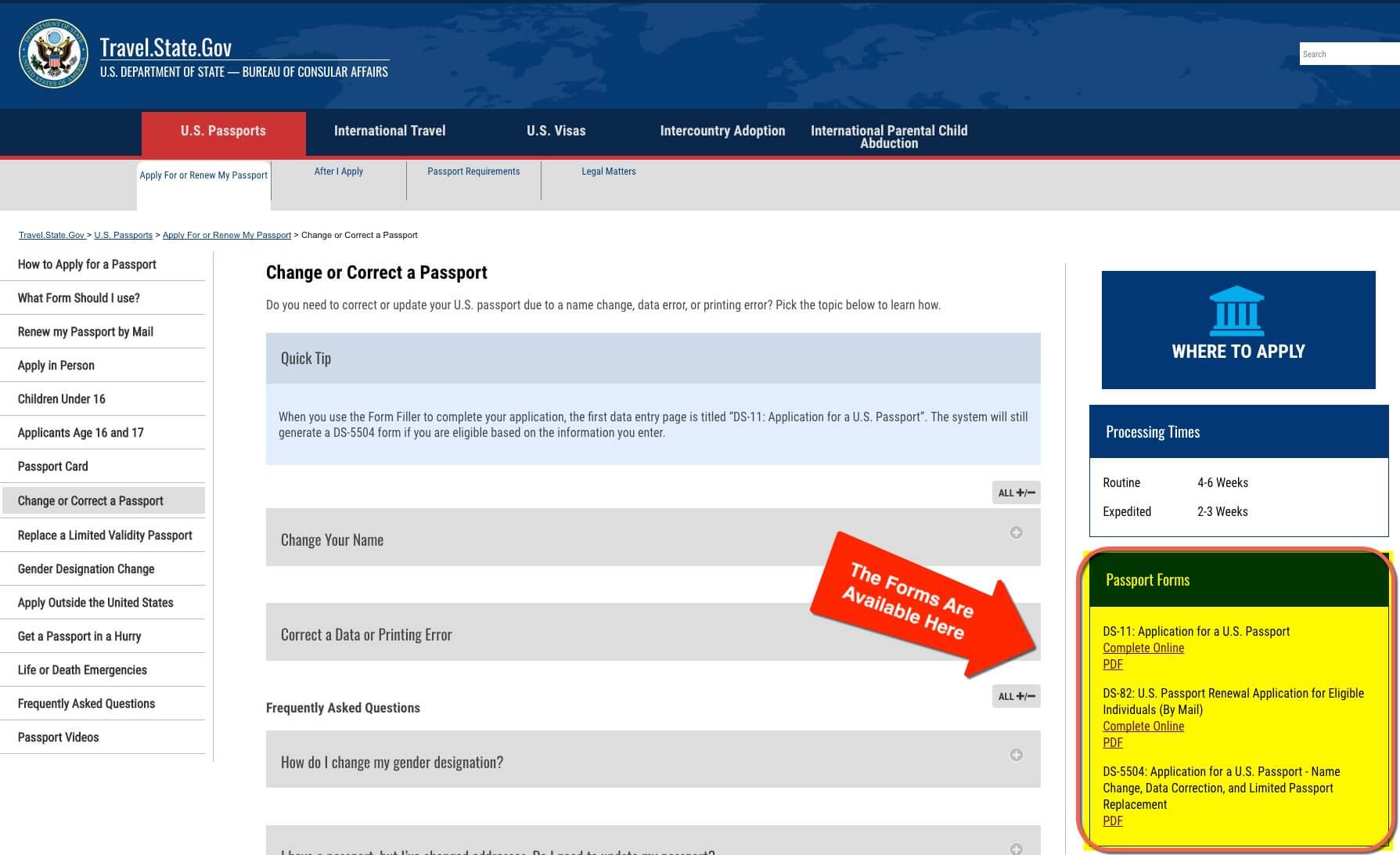This screenshot captures the homepage of the U.S. Department of State's travel website, travel.state.gov. At the top, a blue banner features a lighter blue outline of global continents, showcasing North America on the left, Greenland to the right, and Europe further to the right. In the upper left corner, "travel.state.gov" and "U.S. Department of State" are displayed in white font next to the department's seal, an intricately detailed eagle.

Directly below this, a darker blue navigation bar presents clickable options: "U.S. Passports," "International Travel," "U.S. Visas," "Inter-country Adoption," and "International Parent-Child Abduction." The "U.S. Passports" section is currently selected.

Further down, a gray bar highlights the "Apply for My Passport" section, which is also selected. On the left side of the page, a vertical menu lists multiple options: "How to Apply for a Passport," "What Forms Should I Use," "Renew My Passport by Mail," "Apply in Person," "Children Under 16," "Applicant Age 16 and 17," "Passport Card," and "Change or Correct a Passport." "Change or Correct a Passport" is the currently selected option, suggesting the user's interest in modifying their passport information.